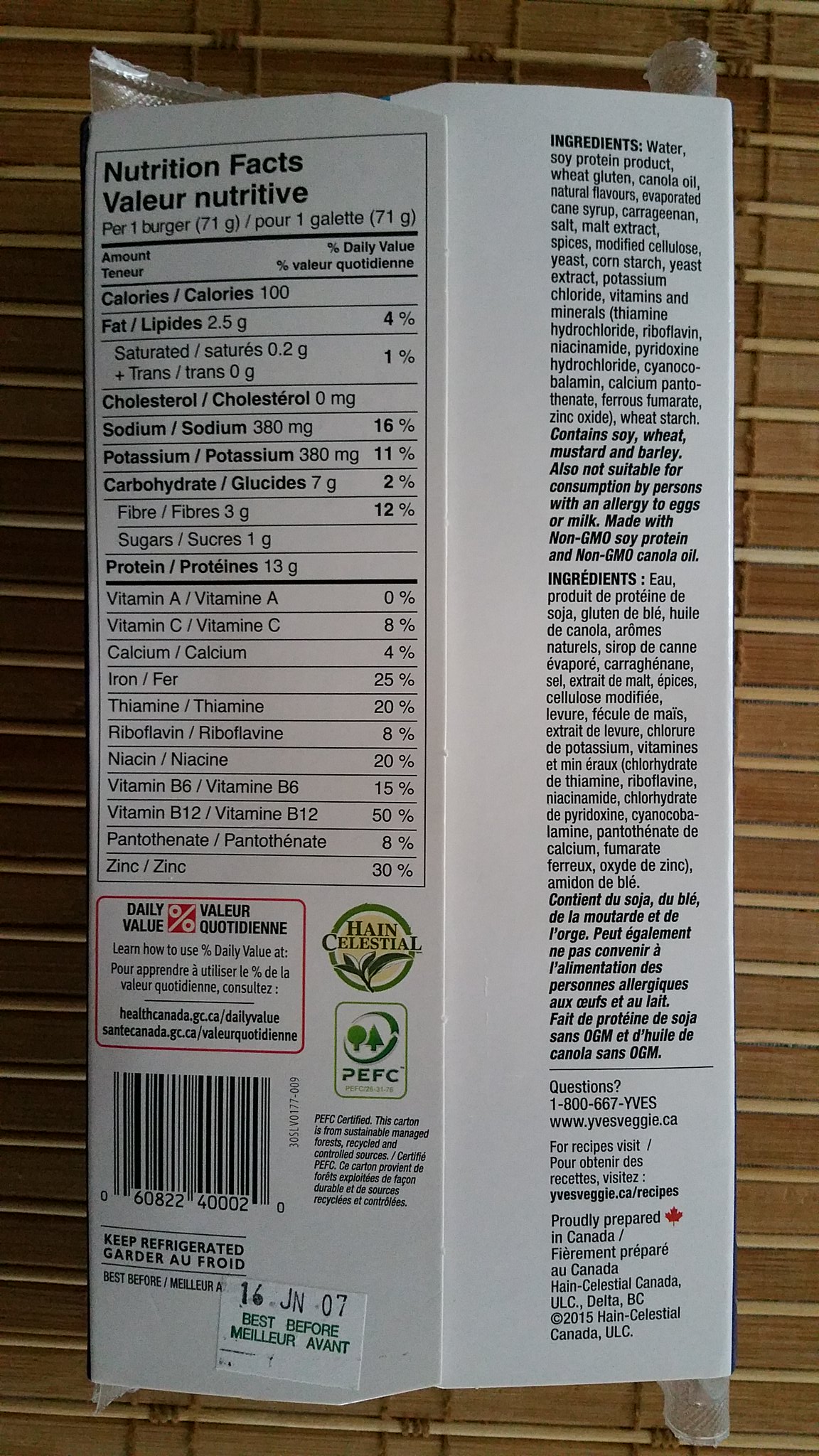The image depicts the back of a white cardboard box of food, featuring nutritional and ingredient information. The background consists of a brown surface, transitioning from dark to light shades. The nutritional values are prominently displayed in a large rectangle with a black border on the top left portion. This section indicates a serving size with 100 calories, 2.5 grams of fat, 380 milligrams of sodium, and 380 milligrams of potassium. Below this, a red square contains black writing regarding daily values.

A notable logo with a green border, yellow background, and a leaf inside reads "Hain Celestial." Adjacent to this logo is another smaller square with the "PEFC" logo, depicting two trees. Further down, the packaging has instructions to keep refrigerated and the text "Gardea or Freud."

The right side of the packaging lists ingredients in both English and French. At the bottom right, there are contact details, including a phone number (1-800-667-EVS) and information on where the product was prepared, signified by a red leaf indicating it was proudly prepared in Canada. Additionally, there is a "Best Before" sticker and a barcode on the lower section of the left side of the image. The detailed information is provided to inform consumers about the product and how to contact the company for any inquiries.